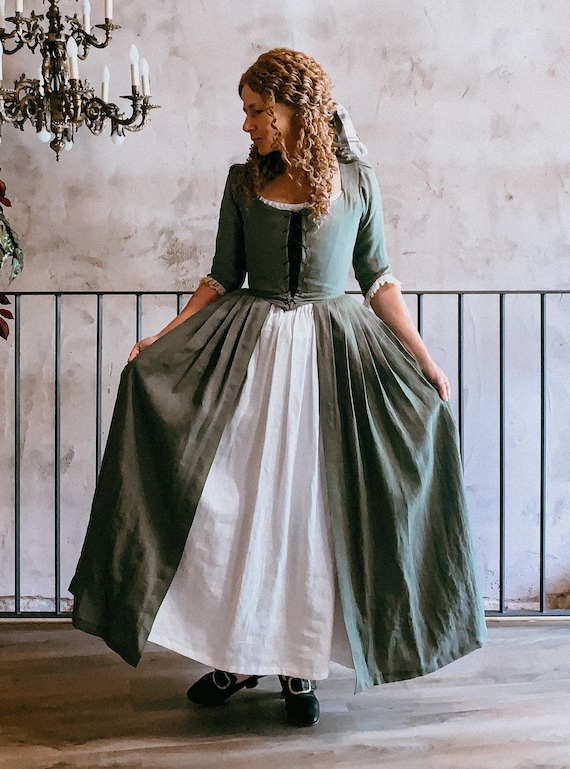The photograph features a young woman dressed in a historical period costume, possibly from the 1600s or 1700s. She is posed holding the sides of her green skirt, which is open to reveal a white underskirt, and she's gazing off to her right, presenting her profile. The dress has a scoop neck and elbow-length sleeves adorned with lace, and it features a laced bodice and wide pleated skirt, possibly made of muslin or cotton. She stands in a setting with an old wrought iron railing behind her and an antique chandelier visible in the upper left corner. The woman has long, curly blonde hair and wears black shoes with silver buckles.